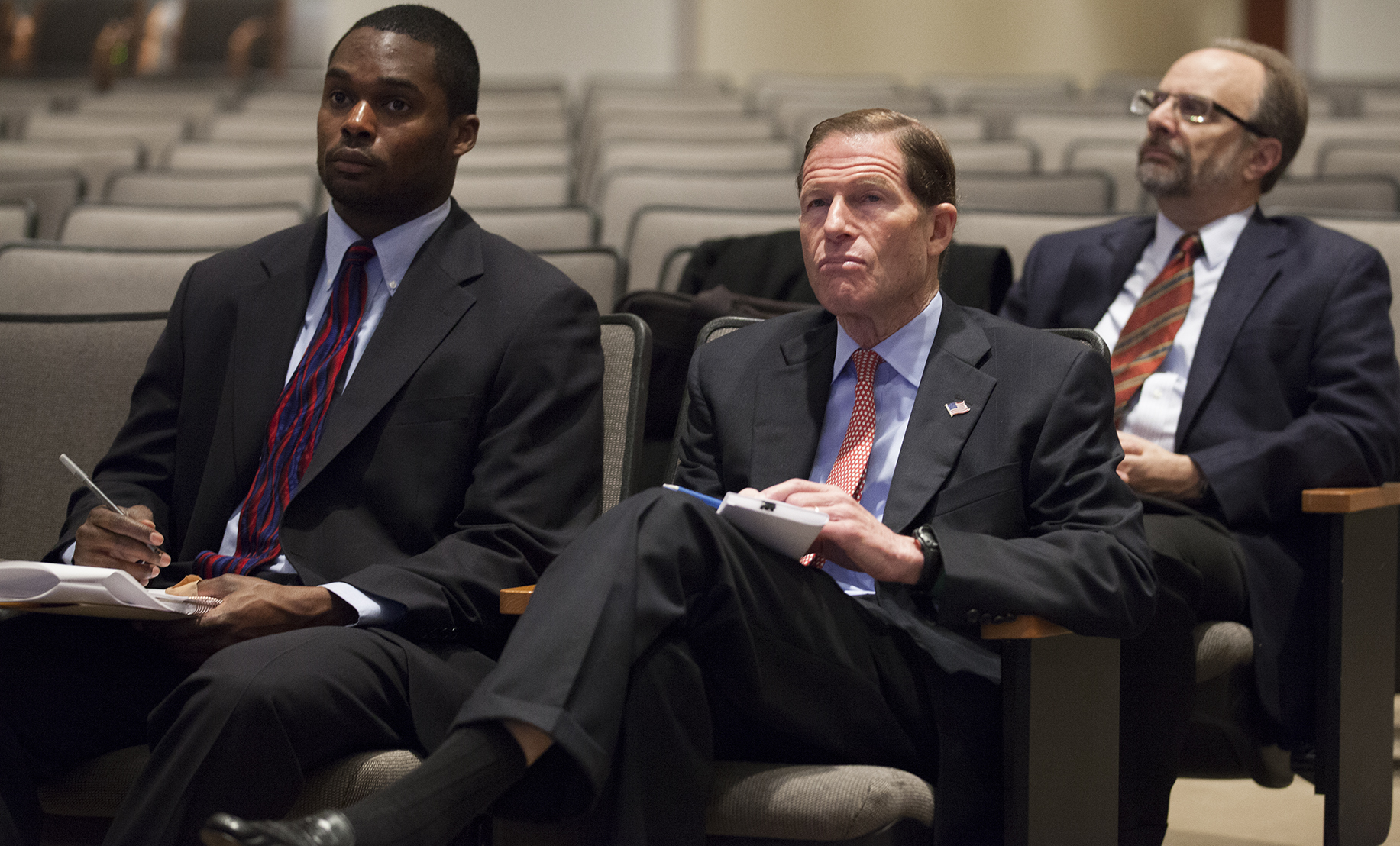This detailed image captures three men seated in an auditorium, possibly at a university event. They are dressed in dark suits, each with distinct accessories and expressions of focus. In the foreground, two men sit side by side. The man on the left, an African American gentleman, sports a blue suit, a blue dress shirt, and a red and blue tie. He is engrossed in writing on a stapled notepad with a pen, which he holds in his right hand. Next to him, a white gentleman is dressed in a dark suit, a blue button-down shirt, and a red tie. He features an American flag pin on his lapel and wears a watch on his left wrist. This man has his left leg crossed over his right, and also seems to be taking notes. 

Behind them, a third man sits alone, wearing a dark blue suit, a white dress shirt, and a red tie with diagonal stripes. He has a square-shaped pair of glasses, a receding hairline, and a goatee, adding to his distinguished appearance. The seating in the auditorium features gray-padded backs and seats, with wooden armrests painted black, enhancing the formal setting. All three men appear to be attentively listening to a speaker or lecturer, indicative of an engaging and important event.